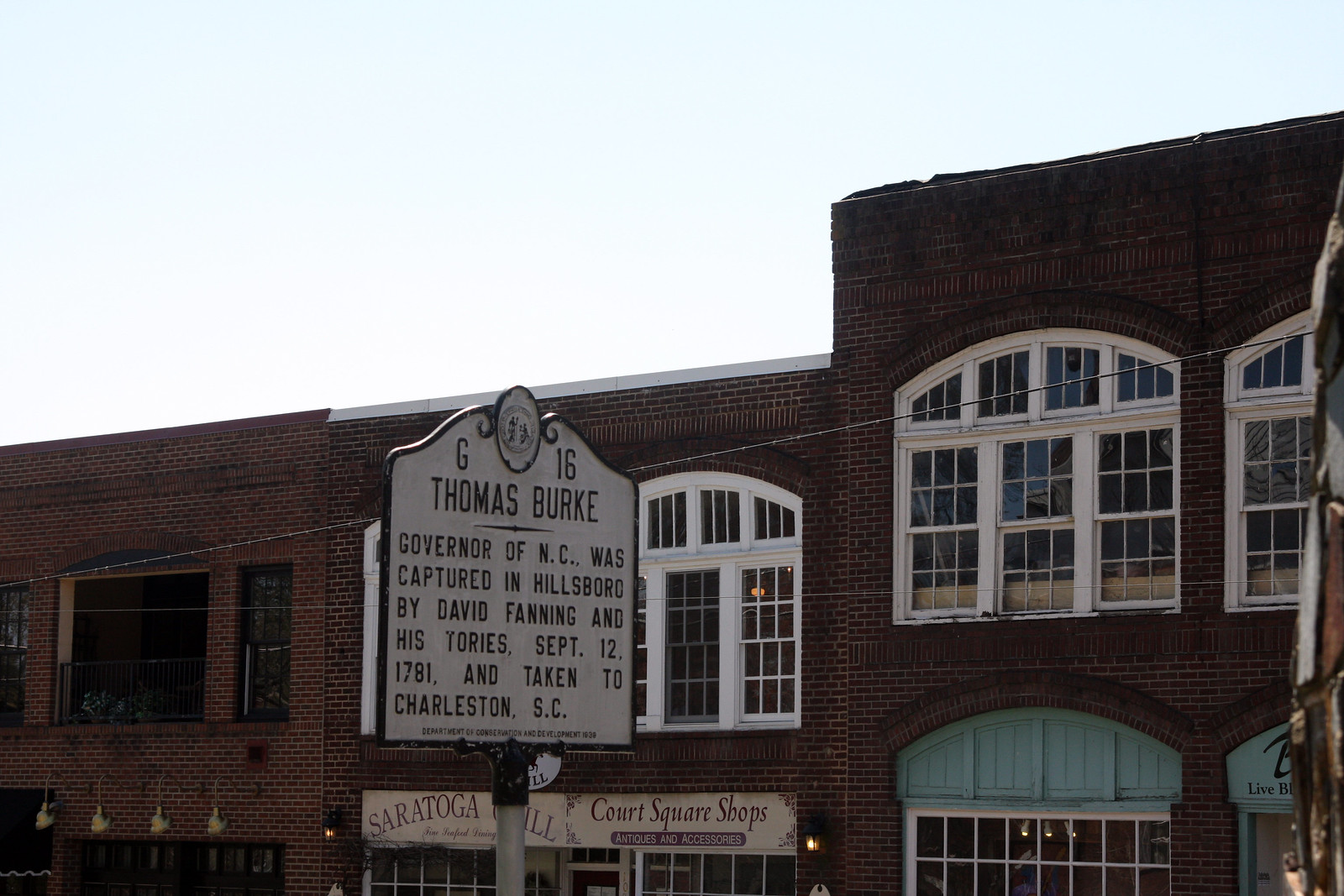The photograph captures a bright, clear day, showcasing a red brick building with two levels of windows, each framed with white borders. The light blue sky serves as a backdrop, enhancing the vividness of the structure. This building, consisting of three sections, becomes slightly higher towards the right, with the left section featuring a large central window and some lighting fixtures on the lower level. Prominently displayed on the facade are signs reading “Saratoga…” and “Court Square Shops, Antiques, and Accessories,” both partially obscured by another sign.

The middle and right sections of the building show signs of aged green paint and wooden framing above some windows. In front of the building stands a historical marker with a white background and black text. The marker reads: 

"G-16. Thomas Burke, Governor of North Carolina, was captured in Hillsborough by David Fanning and his Tories September 12, 1781, and taken to Charleston, S.C."

This historical marker, likely located in North Carolina, provides context to the site's historical significance, with an image of a crest or patch above the text, although it's not fully visible.